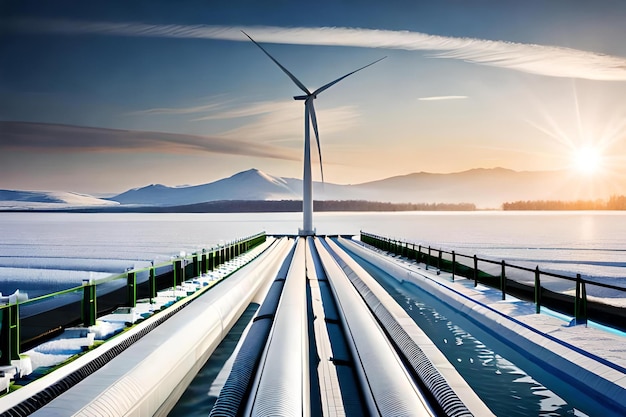The image depicts a detailed rendering of a modern white windmill with three thin blades, situated at the end of a long, straight walkway that stretches across what appears to be a frozen or snow-covered body of water. The scene is framed by a striking background featuring a long mountainous range with snowy peaks, and above it, a sky that transitions from a darker blue on the left to a lighter, sunlit hue on the right. There is an impression of a cloud trail cutting across the sky from left to right. Snow blankets the walkway leading to the windmill, emphasizing a cold, wintry atmosphere. The setting sun, positioned just above the horizon to the right, casts its light across this serene landscape, suggesting a time near dusk. This painting skillfully combines elements of nature and technology against a backdrop of tranquil yet dramatic scenery.